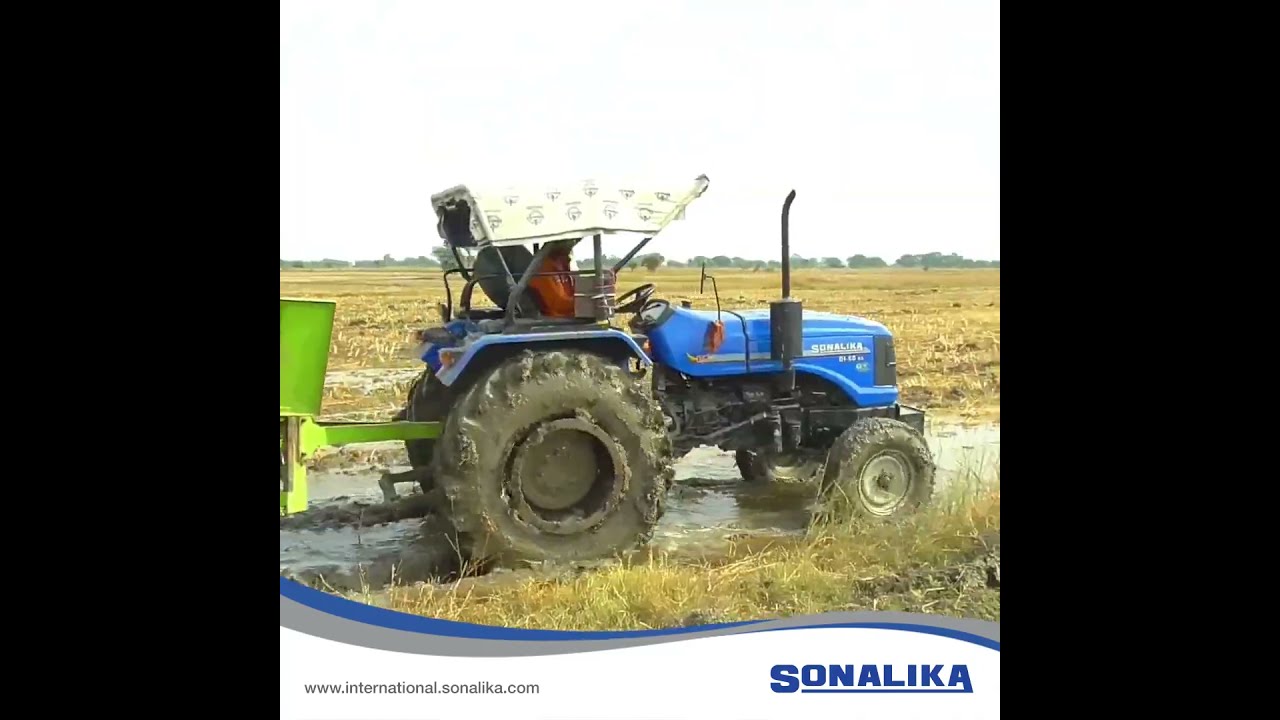The image showcases a vibrant blue Sonolica tractor actively navigating through a muddy and weed-filled field, likely a farm setting. The tractor is fitted with a cream-colored shade canopy over rebar reinforcements, providing protection from the elements. Notably, the canopy features a repeated logo pattern. The tractor, which has large wheels at the back and smaller ones in the front, drags a lime green attachment behind it, indicating that it is in active use, possibly for some farming work. Vertical two-inch black bars frame the image on both the left and right sides. At the bottom, there is a scrolling border effect featuring the Sonolica brand logo and the website www.international.sonolica.com, with the brand name "Sonolica" prominently displayed in blue lettering to the right. The tractor's tires are visibly muddy as it moves through what appears to be an irrigation or drainage canal area, underscoring the functional and rugged use of this farming equipment.